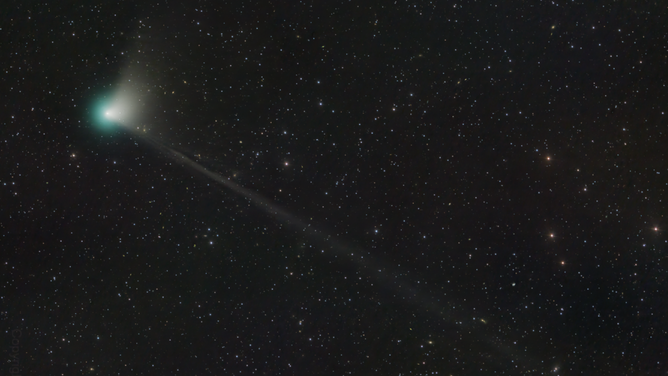The image depicts a vast, dark expanse resembling outer space, likely computer-generated. It is dominated by myriad tiny points of light representing stars and other celestial bodies. Most stars are white, but there are also noticeable blue, red, and light purple hues scattered throughout, along with at least 20 or 30 prominent amber stars. Towards the left-hand side of the image, there is a striking feature: a bright, white light at its core, surrounded by a soft, glowing halo. This halo transitions into a greenish hue, suggesting a resemblance to a comet or asteroid. A diagonal beam of light extends from this radiant center, stretching across the image from the top left to the bottom right, enhancing the overall science fiction ambiance. The stars vary in brightness and size, contributing to the richly detailed and immersive cosmic scene.